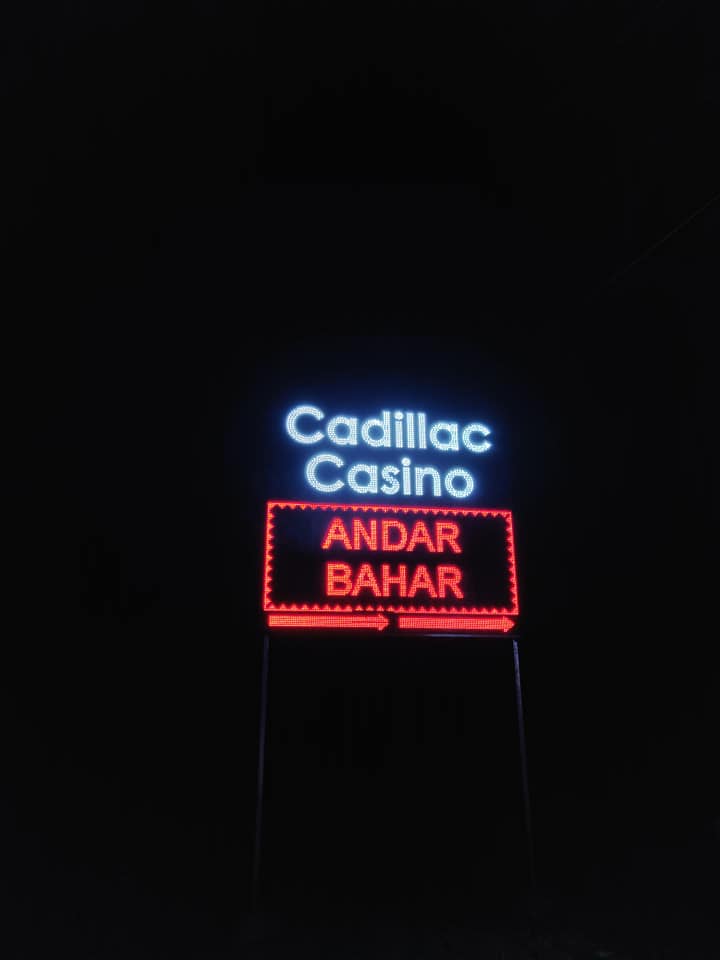In this night-time photograph, the entirely black background is punctuated by a striking neon sign in the center. At the top, a glowing blue neon sign spells out "Cadillac Casino," with a subtle suggestion of off-white hues blending into the light. Beneath this, a vivid red neon rectangular box encloses the illuminated text "Andar Bahar." This red sign is bordered by an LED light and is accentuated by two rightward-pointing arrows, also in red neon, suggesting direction. The entire sign assembly is suspended, likely supported by metal spikes faintly visible against the darkness. The vibrant lights of the Cadillac Casino and Andar Bahar signs create a sharp contrast against the void of the night.